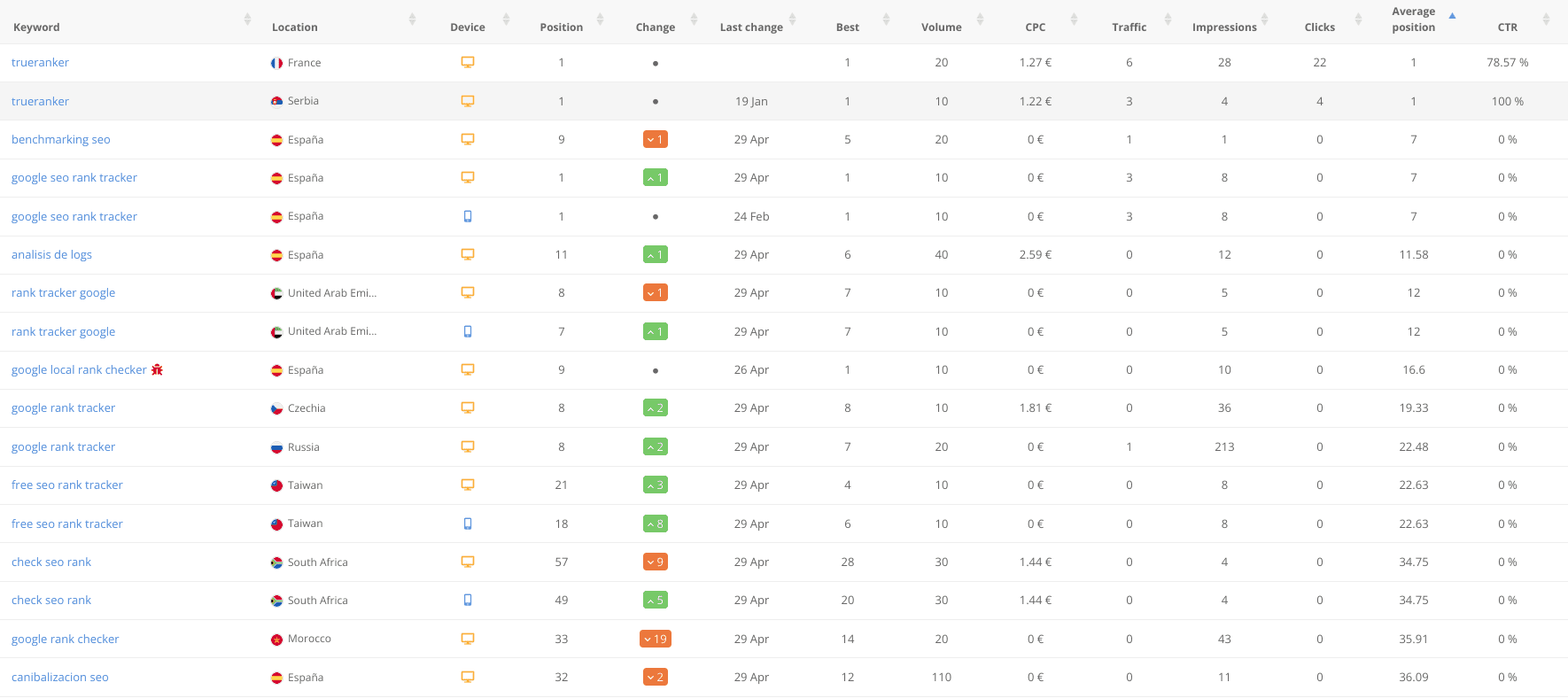This image displays a detailed screenshot of a keyword tracking spreadsheet. The document is organized with a clean, white background, and a very light gray header row at the top, which contains the titles of each column. On the far left, the first column is titled "Keyword," and it lists various keywords in blue font, though the text is quite small and difficult to read. Some identifiable keywords include "Google SEO rank trader" and "check SEO rank."

The spreadsheet extends horizontally with multiple columns that track various metrics associated with each keyword. These columns, in order from left to right, include:

- Location
- Device
- Position
- Change
- Last Changes
- Best
- Volume
- CPC (Cost per Click)
- Traffic
- Impressions
- Clicks
- Average Position
- CTR (Click-Through Rate)

Each column is populated with numerical data corresponding to the respective keyword's performance across these metrics. Despite the small font size of the keywords, the structure and intent of the spreadsheet are clear, showcasing a comprehensive keyword performance analysis tool.